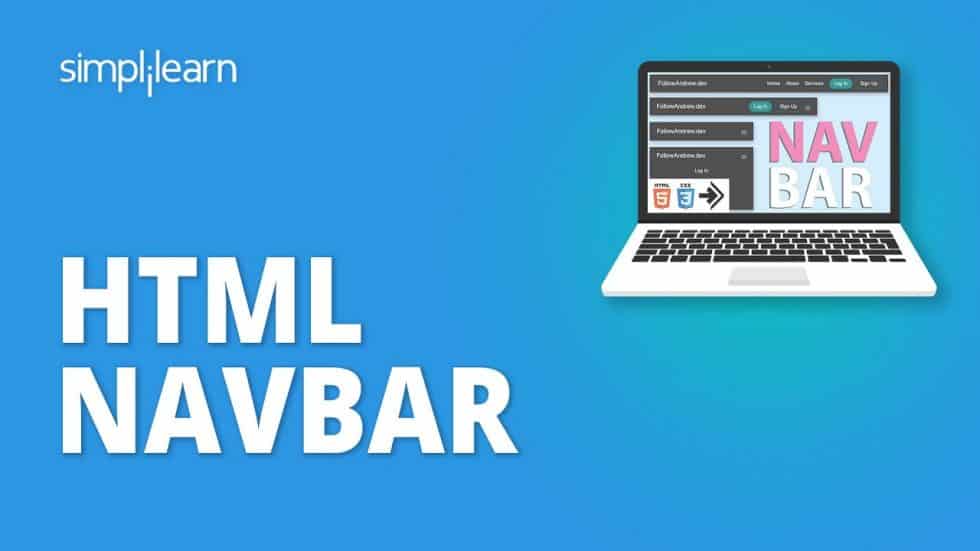The image depicts a blue-themed graphic with several prominent elements. In the upper left corner, the phrase “Simply Learn” is displayed prominently, though the letter 'I' appears slightly misaligned or descending below the baseline. On the bottom left, there is text that reads “HTML Nav Bar.”

On the right side of the image, a laptop is featured with a notable blue background. The screen of the laptop shows the words "Nav" in purple and "Bar" in white, indicating topics related to navigation bars in HTML. The laptop itself has a white keyboard with black keys. Additionally, a subtle white hue accentuates the top right behind the laptop, adding depth to the background. 

There is also a green button visible in the image, suggesting interactivity or a clickable element. The overall composition places emphasis on educational content related to HTML and navigation bars, enhanced by the blue and white color scheme.